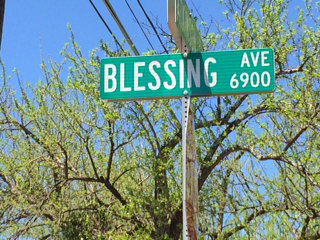This outdoor photograph features a street sign that reads "Blessing Avenue 6900" in white block letters on a green rectangular background. The sign is affixed to a metallic stake characterized by thin, layered strips for structural integrity and holes running down its side. An additional street sign is mounted above, extending in the opposite direction, though its text is obscured. Beneath these signs is a stop sign. The image captures a vibrant blue sky and a large tree in the background, indicative of springtime with its bright green buds on sprawling branches. Electrical wires diagonally traverse the scene, running from the bottom right to center left, further enhancing the outdoor setting's dynamic quality.